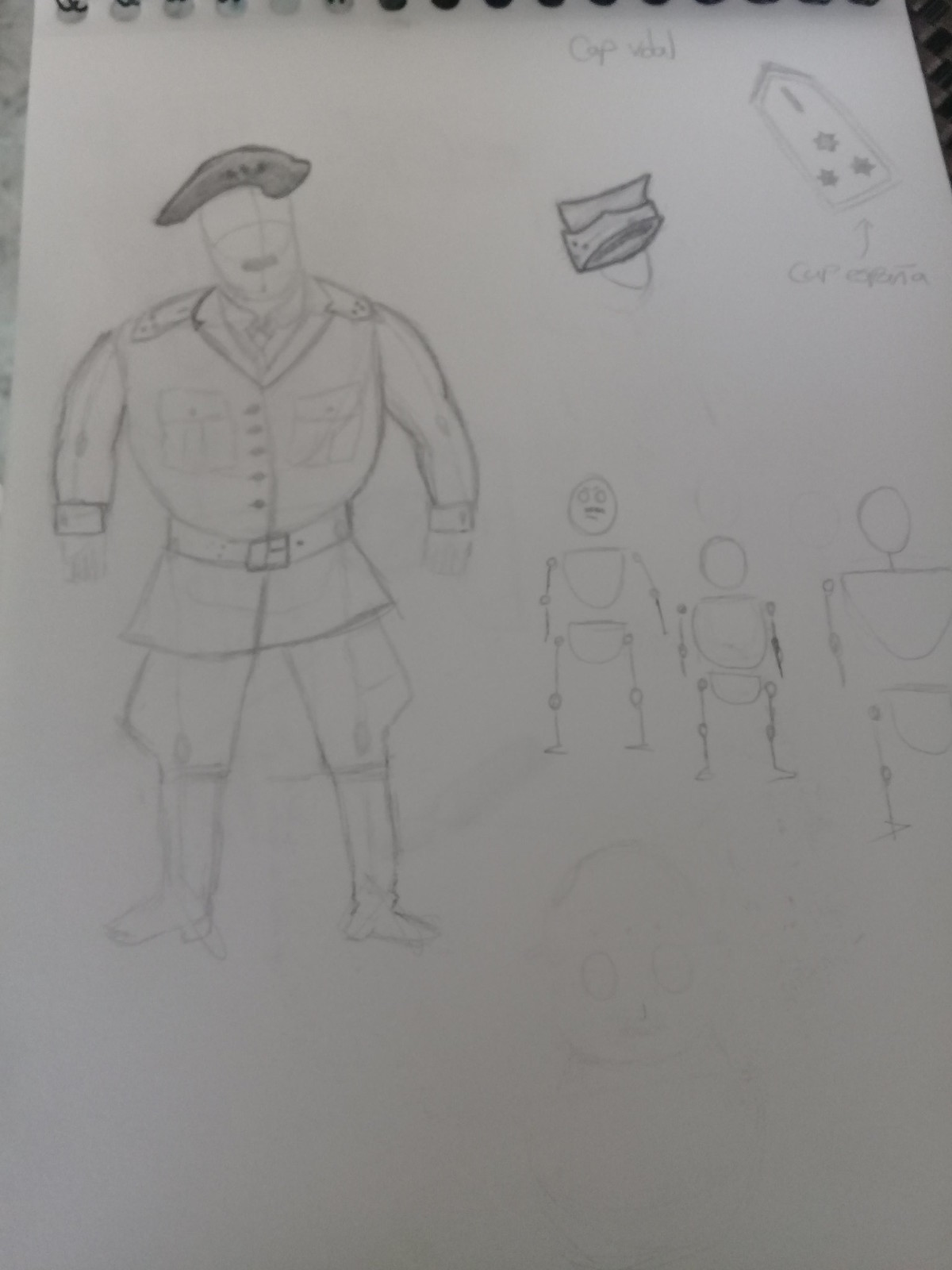This image, a child’s pencil drawing on a white notebook page with visible metal rings at the top, depicts a detailed scene centered around a military figure. On the left side of the page stands a large man, distinguished by his broad chest and broad shoulders, dressed in what appears to be a military uniform. He wears a dark beret and a coat-like jacket with patch pockets, buttons, and a belt around his waist. His uniform also includes epaulets or insignia on the shoulders, a tie, and riding breeches that taper down to tall boots below the knee. His uniform resembles that worn by officers during World War II, providing a historical touch to the drawing. His arms rest at his sides, and his eyes are depicted as closed. To the right of this central figure are three stick-like robotic figures with circular heads, square or diamond-shaped chests, and stick limbs. Only one robot features facial details, with a simple circle and slash for a mouth. Above these robotic figures, there is a drawing of a military cap with a chin strap, and to the right, a detailed emblem or insignia with three stars and writing below it, indicating rank. Despite some faint and blurry areas in the pencil drawing, these intricate details create a vivid portrayal of a military scene as imagined by a child.